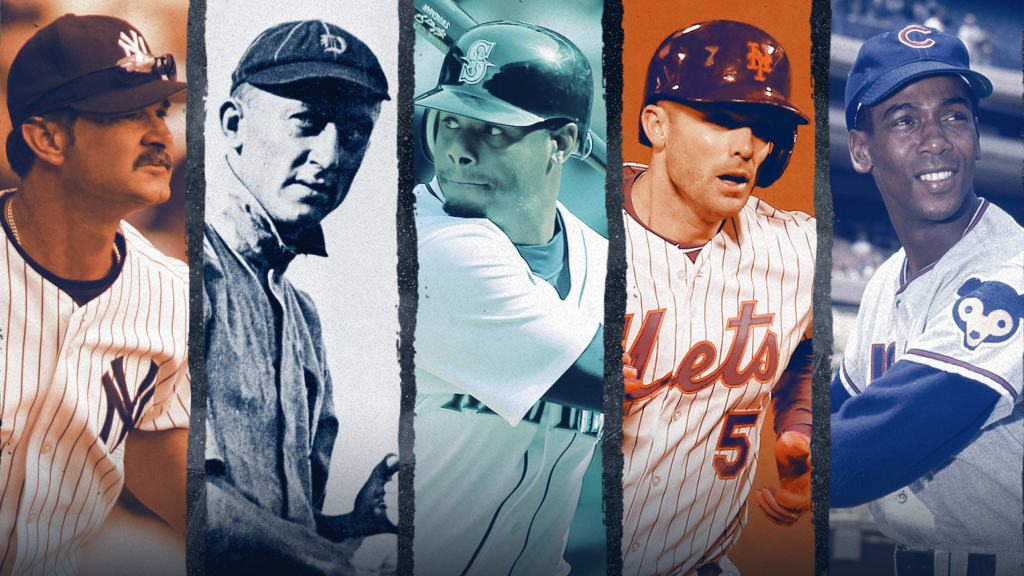The image is a collage of five baseball players, each uniquely tinted except for one, covering various teams and time periods. Starting from the left, the first photo is in a reddish-orange hue, portraying a New York Yankees player. He wears a Yankees jersey with blue pinstripes, a black cap marked "NY" in white, a blue undershirt, and sunglasses perched above his cap. He sports a mustache and is looking right.

Next is a black-and-white photograph of an older-era player with a short, rounded cap. This player wears a clean white jersey, looking directly at the camera, suggesting it might be from a much earlier period.

The third image, tinted cyan, features a player preparing to bat with a black or blue helmet bearing an "S." He has a small goatee, a barely visible mustache, a blue t-shirt under his white jersey, and he holds a black bat over his shoulder. His helmet and jersey indicate he might be from a team with an "S" as an emblem.

The fourth player, in a red-orange tint, is from the New York Mets, as denoted by the "NYM" on his dark blue or black helmet with a face shield. His white jersey has "Mets" and the number 5 written on it, with a long-sleeved blue or black shirt underneath. He is clean-shaven and gazes directly ahead.

The last image features a player with a Cleveland Indians cap, signified by the "C" outlined in white. He is African-American, smiling while looking right, and has the team mascot, a bear, on his shoulder. He wears a white jersey over a dark blue sweatshirt.

In this diverse and historically rich collage, each image captures distinct aspects of baseball's heritage through the uniforms, equipment, and eras represented.